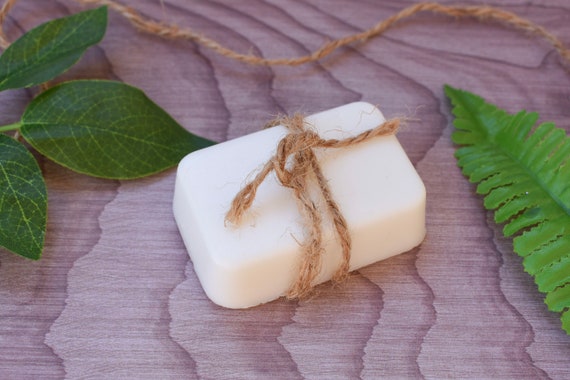This meticulously staged product photograph, ideally suited for an e-commerce website or shopping catalog, features a rectangular bar of white soap with elegantly rounded corners. The soap is adorned with a decorative piece of brown twill rope, wrapped twice around its center and tied into a neat knot at the front. This setup is placed atop a flat, pinkish-brown wooden surface, showcasing its natural streaks of darker brown. The scene is enhanced by additional elements: more twill rope laid out straight above the soap, a long, fur-like green leaf positioned on the right side, and a stem bearing three round, darker green leaves on the left. This arrangement not only highlights the soap but also adds a touch of organic elegance to the composition.